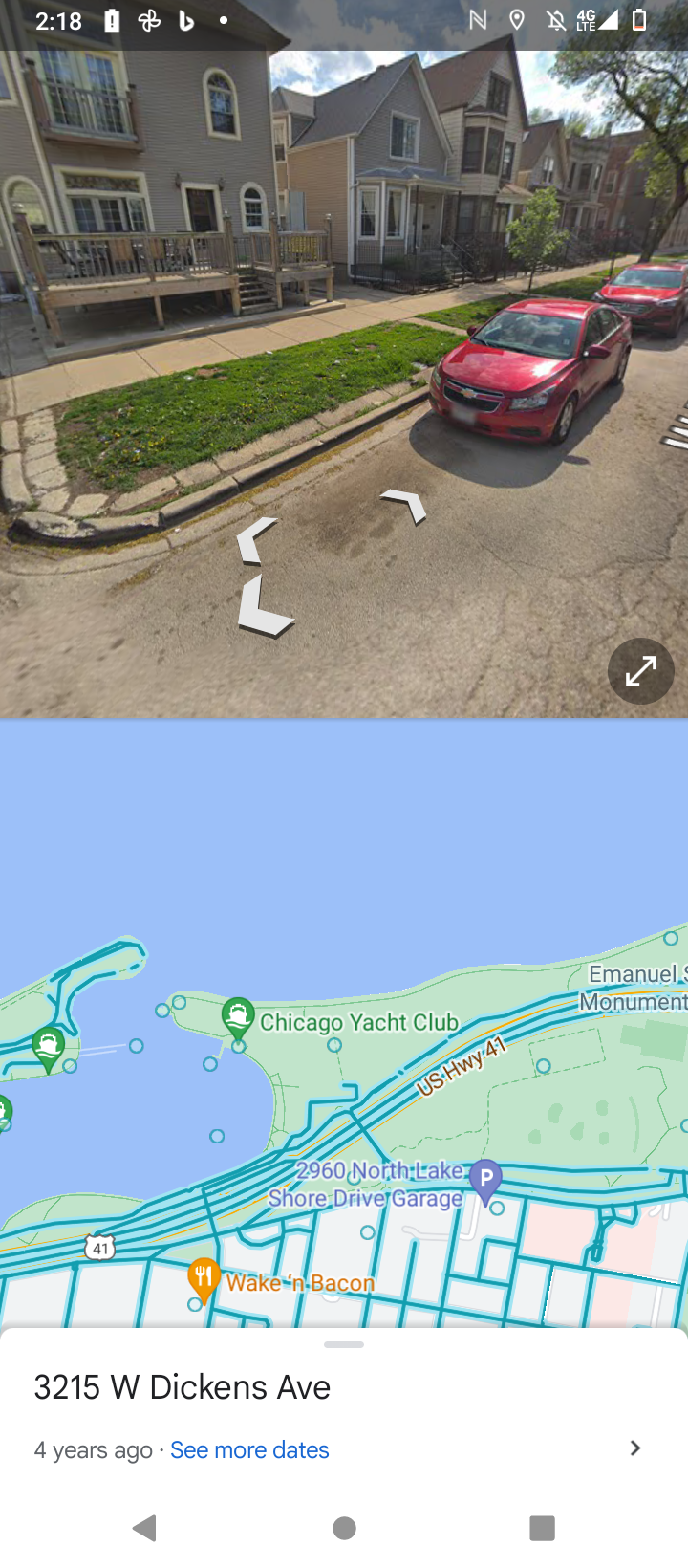The image captures a scene from a doorbell camera, though it also resembles a view from a car's backup camera, complete with white directional arrows indicating parking zones. The upper portion of the image showcases a row of houses. On the right side, there's a gray house with a deck on the bottom floor and a small balcony accessible through two French doors on the top floor. This house also features two distinctive arched windows on the left side, combining a flat bottom with an arched top. A sidewalk and a patch of grass are visible in front of this house. 

Next to it, another house follows with a design that includes one lower peak and one higher peak. The architectural style proceeds similarly down the block. On the left side of the photo, a tree and two red cars are parked by the street. The street is marked with white arrows indicating parking spots in front of the first red car.

The lower half of the image includes a map, suggesting it might be from a vehicle's navigation system. It displays the address "3215 West Dickens Avenue" and nearby landmarks including the Chicago Yacht Club and Wig and Bacon. A monument is noted, alongside a "four years ago" timestamp with an option to "see more dates." The map itself has a blue background representing water areas and green patches for land, with blue lines delineating streets.